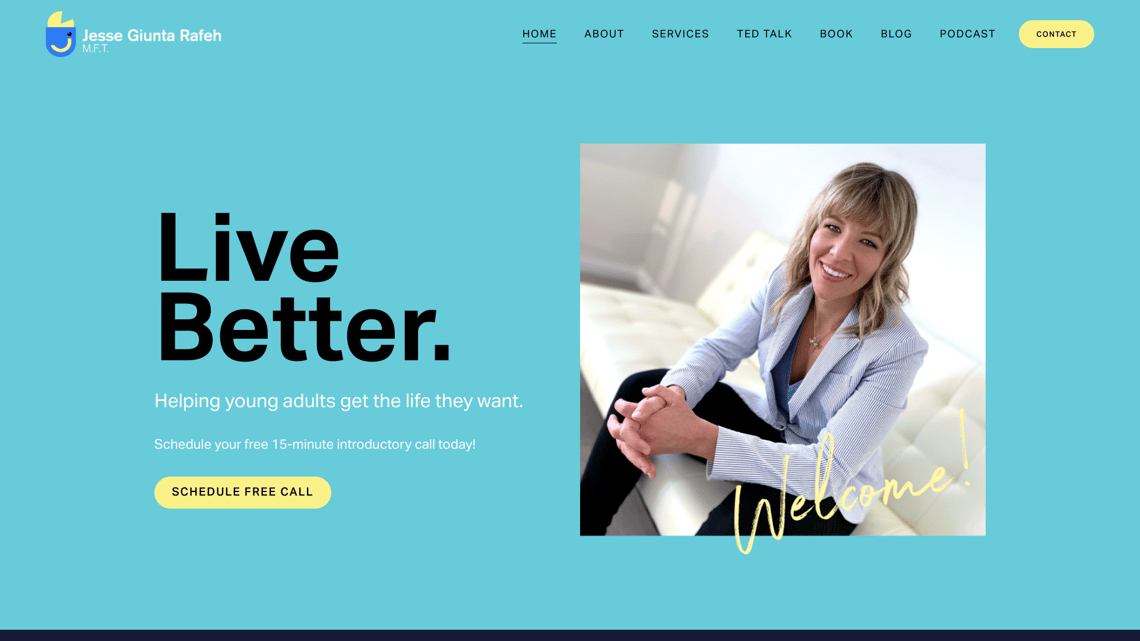The homepage of what appears to be a personal website features a blue logo resembling a basket or a Pac-Man shape. The text "Jesse Guinta Rafe, MFT" is prominently displayed. The navigation menu includes tabs labeled Home, About, Services, TED Talk, Book, Blog, Podcast, and Contact. 

The page has a light green background with black text in the center that reads "Live Better," followed by white text stating, "Helping young adults get the life they want. Schedule your free 15-minute introductory call today." A yellow button below this invites users to "Schedule Free Call."

On the right side of the page is a photograph of a woman, presumably Jesse Guinta Rafe. She appears to be in her forties, with dirty blonde hair, wearing a blazer, necklace, and black slacks. She is seated on a white sofa in a white room, leaning forward with her forearms resting on her thighs. Above the photograph, "Welcome!" is written in yellow, handwritten lettering.